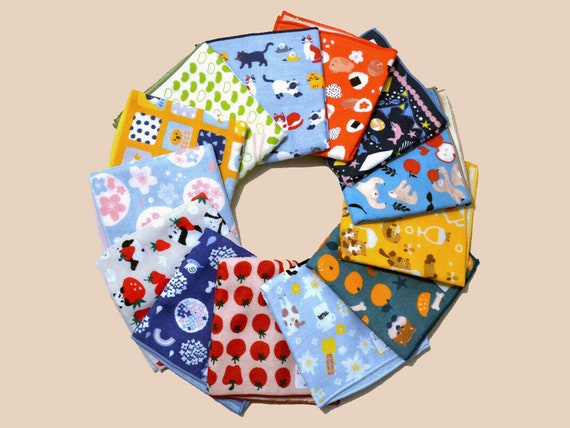The image depicts an arrangement of folded napkins meticulously placed on a plain light pink background. The napkins are organized in a circular pattern, creating a visually appealing composition. Each napkin features a distinct and colorful print. Starting from the top and moving clockwise: 

1. A light blue napkin with a whimsical print of cats.
2. A napkin showcasing a variety of flowers and rocks.
3. A napkin adorned with stars and dolphins.
4. A napkin featuring charming bears alongside other animals.
5. A napkin that boasts a vivid fruit motif, including tomatoes.
6. A napkin decorated with intricate floral patterns.
7. A napkin printed with unique white and gray roundish shapes.
8. Another, a vibrant piece with pandas holding strawberries.
9. A napkin with colorful squares that contain spots.
10. A light blue napkin speckled with daisies and perhaps a cow.

Each napkin contributes its unique design, ranging from playful animal prints and fresh fruits to floral bouquets and abstract shapes, adding to the eclectic and vibrant collection.